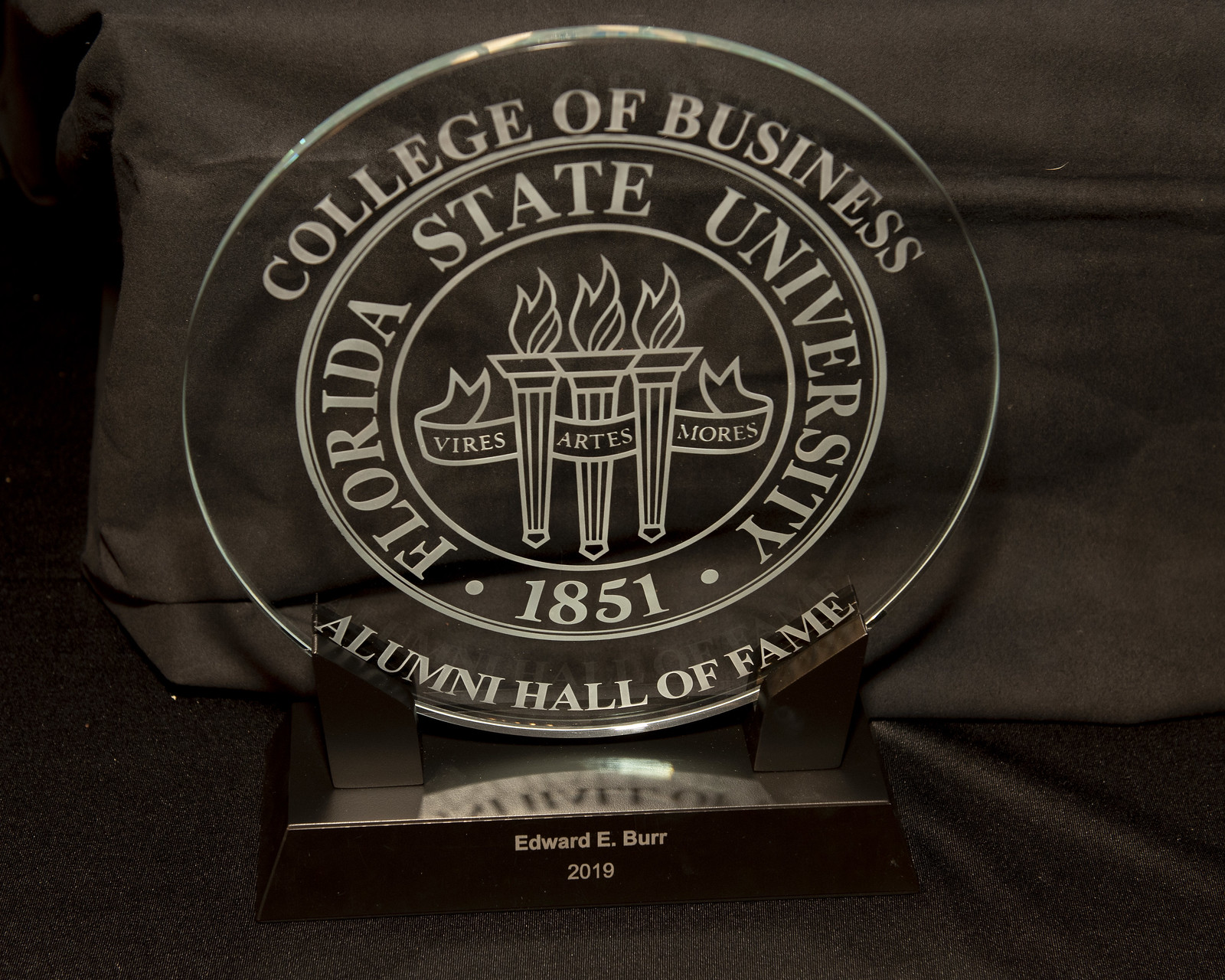The photograph captures a prestigious award featuring a clear circular acrylic piece, prominently displaying white text and a central seal. The award reads, "College of Business, Florida State University, 1851, Alumni Hall of Fame." At the center, there is a logo of three lit torches with a banner that states, "Vires Artes Mores." This transparent circle award is elegantly mounted on a rectangular brown pedestal, which bears the engraved name "Edward E. Burr, 2019." The award is positioned against a dark brown background on a soft surface, with subtle reflections seen on the acrylic.